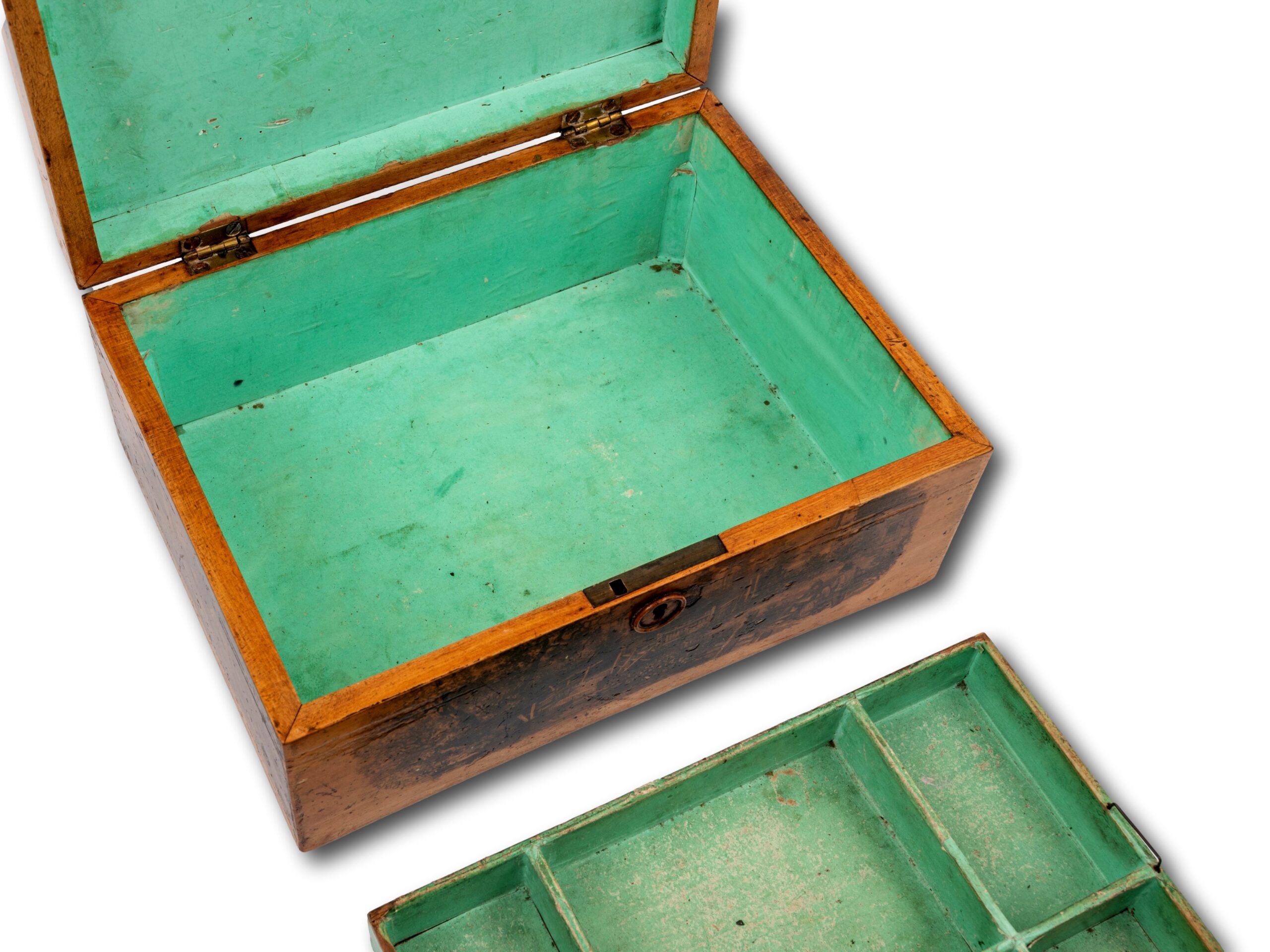This image features an antique wooden box with a rich brown exterior. The box has a lid equipped with two golden hinges, allowing it to open and close. Currently, the lid is open, revealing an interior painted in a mix of lime green and turquoise hues. The paint inside appears old, with signs of wear and possible rust, lending a sense of history to the box. At the front, there is a keyhole, slightly rusty, indicative of its age.

In the foreground, part of another box is visible. This secondary box appears to be painted in the same turquoise color on the inside. It is divided into compartments; two larger sections and at least two smaller ones are visible, suggesting a total of six compartments. While the lid of this second box isn't visible, it is presumed to have one, similarly lockable as evidenced by a keyhole and a possibly concealed latch mechanism.